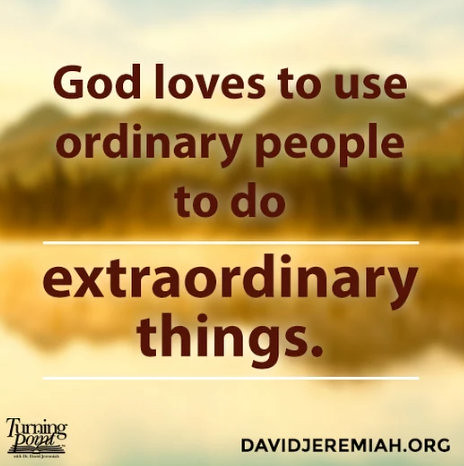The image features a motivational quote that reads, "God loves to use ordinary people to do extraordinary things," with the words rendered in a brown color. The background, while blurred, appears to depict trees with hints of green, brown, and yellow, emphasizing the focus on the quote itself. The setting of the image is bright and clear, enhancing the overall clarity and readability. In the bottom left corner, the text "turning point" is displayed, and in the bottom right corner, there is a website URL, "davidjeremiah.org." This visually appealing image, likely intended for social media, serves as a source of inspiration and encouragement.